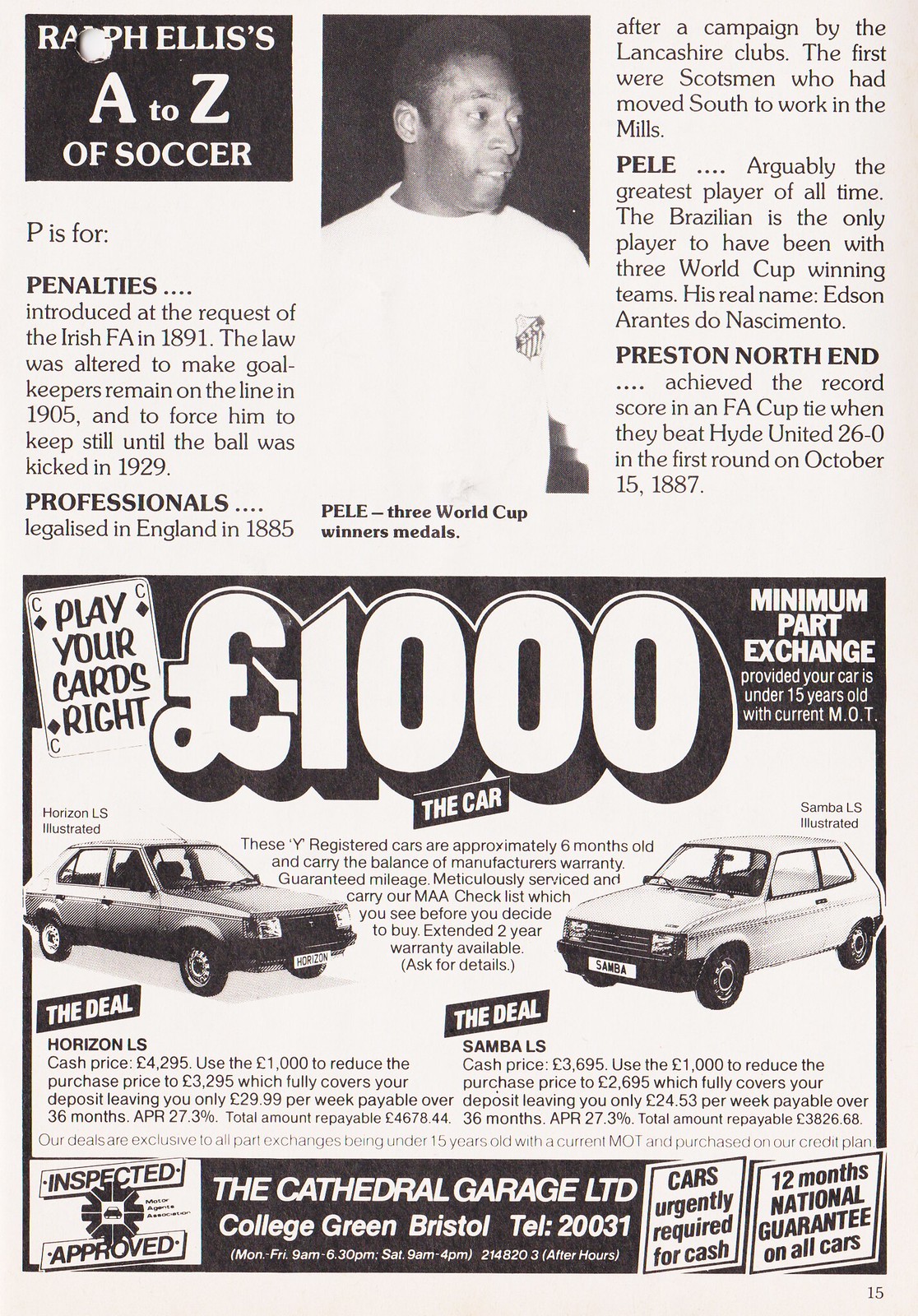The black and white image appears to be a newspaper or magazine article from page 15, titled "Ralph Ellis' A to Z of Soccer." The highlighted section focuses on the letter 'P,' covering various soccer-related topics. It states that penalties were introduced at the request of the Irish FA in 1891, with subsequent changes in 1905 and 1929 regarding goalkeeper movement. The article also touches on the legalization of professional players in England in 1885 after efforts by Lancashire Clubs, noting that the first professionals were Scotsmen who moved south to work in the mills. It includes a section on Pelé, lauding him as arguably the greatest player of all time and mentioning his unique achievement of being on three World Cup-winning teams, with his full name given as Edson Arantes do Nascimento. Additionally, it discusses Preston North End's record-setting 26-0 FA Cup victory over Hyde United on October 15, 1887. In the center of the page is a photograph of Pelé, and at the bottom, there is an advertisement featuring several cars, possibly unrelated to the main soccer content.